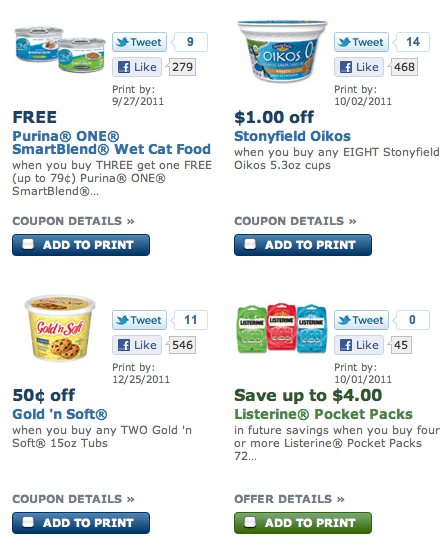The image displays a collection of food and product listings with promotions and offers. 

1. **Free Smart Blend Wet Cat Food**: A promotional deal where you get one item free when you purchase another, with a maximum value of $0.79.

2. **$1 Off Stonyfield Oikos Yogurt**: Receive a $1 discount when you buy any eight Stonyfield Oikos 5.3-ounce cups.

3. **$0.50 Off Golden Soft Margarine**: Save $0.50 when you purchase any two Golden Soft 15-ounce tubs.

4. **Save Up to $4 on Listerine Pocket Packs**: Future savings of up to $4 when you buy four or more Listerine Pocket Packs.